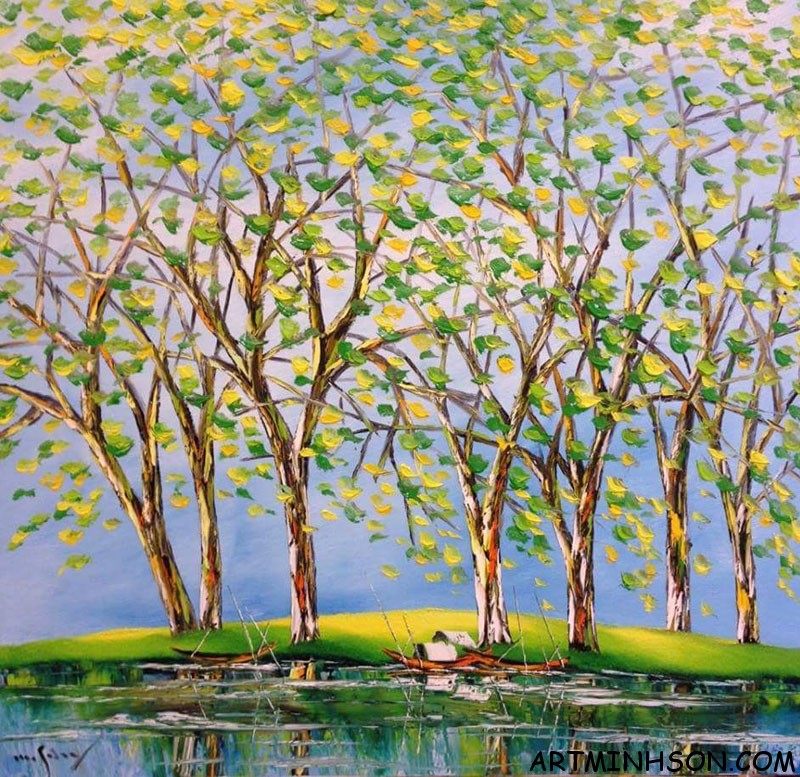This contemporary painting showcases a cluster of thin-trunked trees with branches interwoven in a lace-like pattern, adorned with an array of green shades, from lime to dark green and hunter green, interspersed with yellow leaves. The trunks and branches exhibit a blend of brown and white hues. The trees are perched on a small grassy mound, which is bordered by water, creating reflective ripples that mirror the trees. Scattered pieces of bark are visible at the base of the trees. The backdrop features a gradient sky, transitioning from lighter blue at the top to darker near the horizon. In the bottom right corner, "artmensun.com" is inscribed in black text. The overall composition exudes a sense of serene natural beauty.